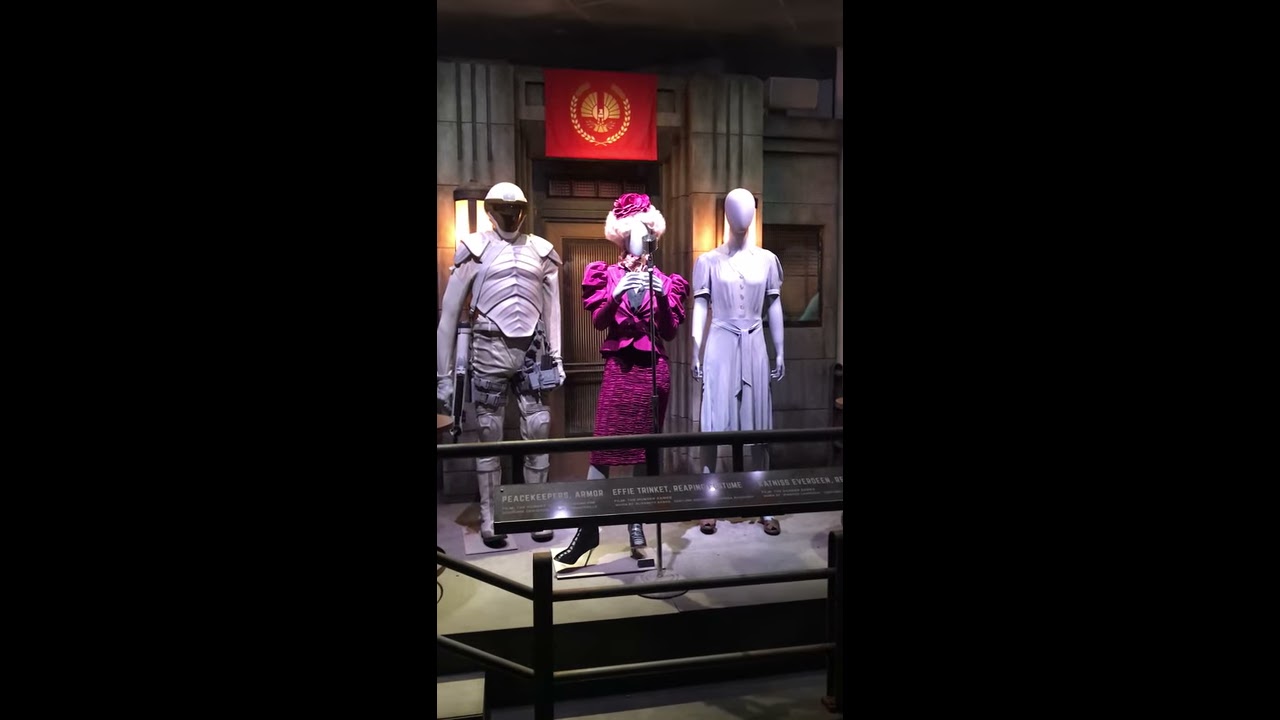The vertically-framed cell phone image appears to be a screenshot from a video game set in an indoor environment resembling a museum or a government building, with distinctive gray stone walls. It shows three robot-like characters standing on a platform, each in different outfits, distinguished by blank faces and without any facial features. Central to the scene, the middle robot is dressed in a striking pink dress reminiscent of the character Effie Trinket from The Hunger Games, known for her extravagant outfits. To the right is a character seemingly dressed in an outfit similar to Katniss Everdeen's District 12 attire, while the left character appears to be clad in what looks like a Peacekeeper uniform from the Capitol. Above the robots, a red flag adorned with a central gold insignia is displayed, echoing the insignias from the Panem universe. The exhibit is visually framed with black bars on either side, and the scene is clearly set up behind a railing, suggesting these are mannequins or models on exhibit, possibly authentic costumes from The Hunger Games series, displayed in a museum-like setting for visitors to view.